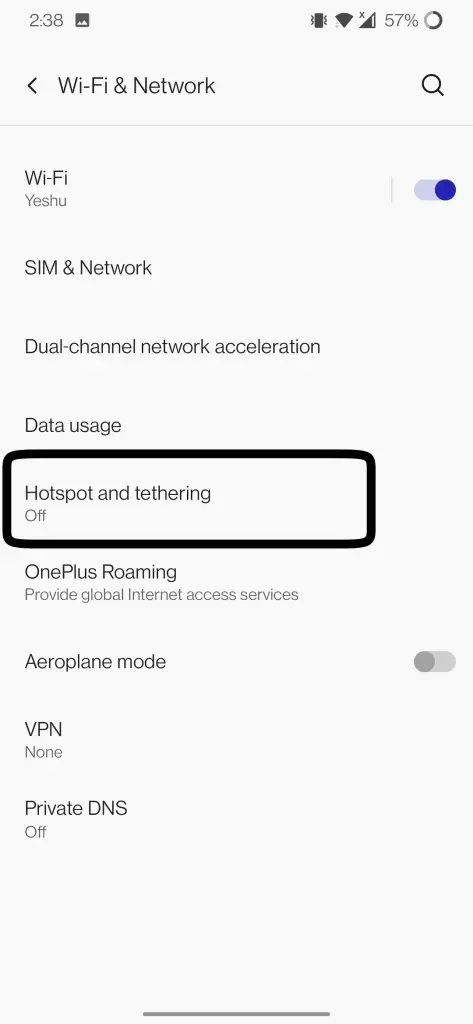This screenshot, captured on a tablet or smartphone at 02:38 (military time), depicts various system and network settings. 

In the top status bar, a few icons are visible:
- A small silhouette of a mountain on the left.
- An icon on the right indicating the device is set to vibrate, a full Wi-Fi signal, and an almost full cell phone signal with an 'X' above it, signifying no SIM card is installed.
- The battery percentage is shown as 57%, and beside it, a circular icon halfway filled, perhaps indicating an ongoing refresh or installation process.

Below these icons, the settings interface displays several options:
- At the top of this section is a back arrow labeled "Wi-Fi and networks." On the right is a magnifying glass icon for search.
- The first setting is "Wi-Fi," which appears to be enabled, as indicated by the gray text "yeshu" slid to the right.
- Below that, the "SIM and network" settings are shown with obscured text "T-E-R M-A-R-I" overlaying this section.
- A section for "Dual Channel Network Acceleration" follows.
- The "Data issues" section is next in line.
- The "Hotspot and tethering" option is set to "off" with a thick black rectangle.
- "OnePlus Roaming" is listed, described in gray text as "provide global internet access services."
- "Airplane mode" and "VPN" settings follow, where VPN is stated as "none."
- Finally, "Private DNS" is noted to be disabled.

The bottom of the image includes a watermark stating, "This image is protected."